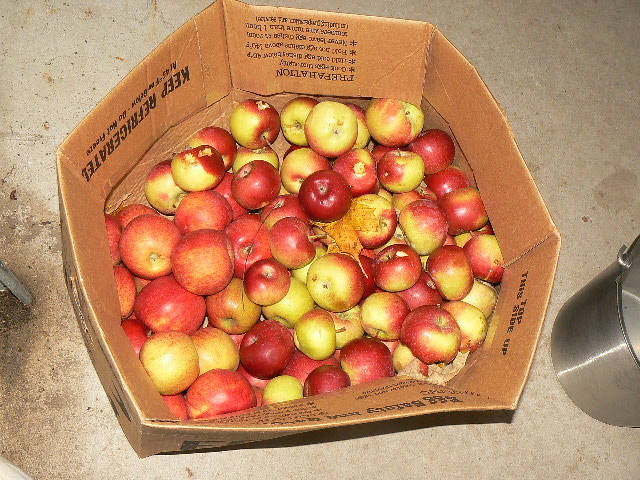This vivid photograph captures an overhead view of a well-worn, five-sided cardboard box filled with apples, placed on a concrete floor. The box, slightly misshapen from extensive use, is folded inward at the flaps and shows signs of slumping. The apples inside, numbering around three dozen, display a variety of colors—ranging from solid red to shades of red and yellow, evoking the appearance of freshly picked fruit from an apple tree. The scene is completed by the presence of a large leaf among the apples and a metal bucket positioned to the right, partially resting on the box and extending onto the concrete surface.